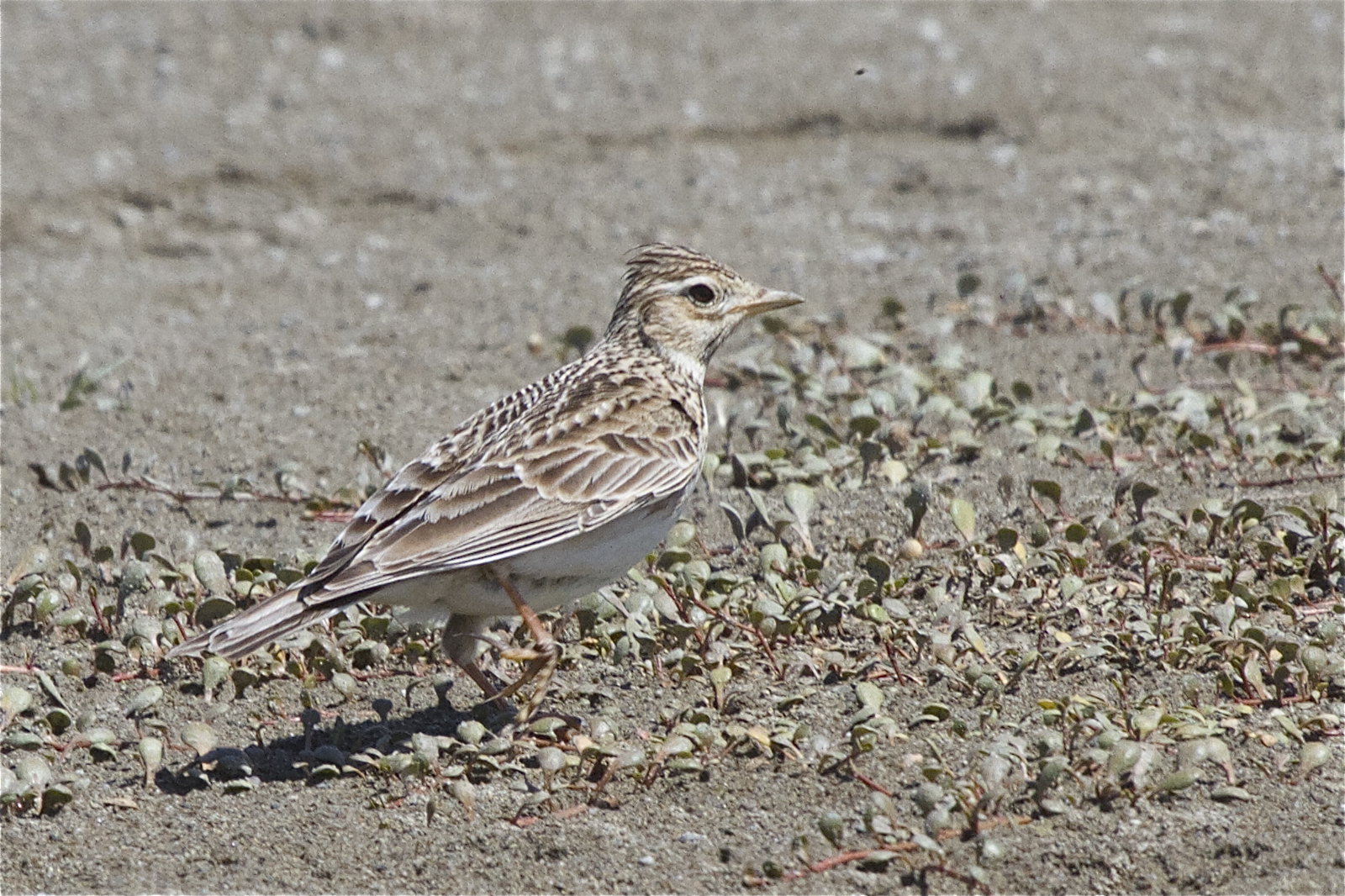This color photograph, taken outdoors on a bright, sunny day, features a charming small bird caught mid-walk on a stark, sandy landscape. The ground, composed of dirt, sand, and gravel with scattered patches of small green plants, is tinted in shades of beige and tan. The bird, positioned almost in the center of the image, is shown in a side profile facing right, with its right leg raised as if it were taking a step. Its plumage—consisting of a blend of brown, beige, and white feathers—provides excellent camouflage against the earthy background. The bird's striking features include a small, pointed beak, a medium-sized black eye, and white feathers on its chest and underbelly. The scene is devoid of other animals, people, trees, or water, highlighting the bird as the sole subject in this serene and minimalist setting.